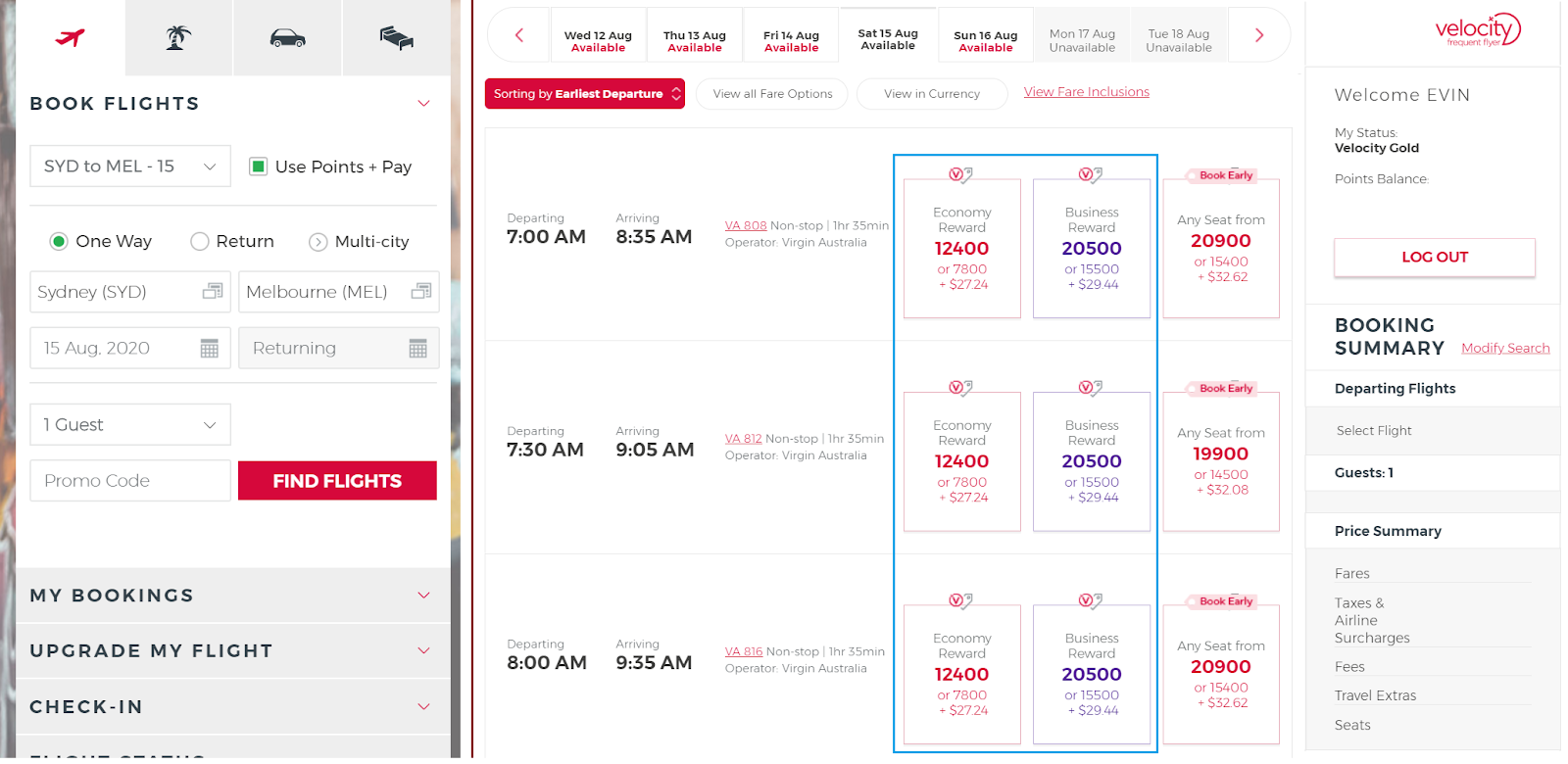**Detailed Caption for Image of Flight Booking Webpage:**

The image depicts a flight booking webpage with a layout designed to facilitate easy navigation and booking management. On the left-hand side, there's a prominent header reading "Book Flights" accompanied by a red airplane icon. Below this header, users are informed of the option to "Use Points Plus Pay" in an illuminated green box.

The itinerary currently displayed is for a one-way trip from Sydney to Melbourne for one passenger, with the date clearly specified. A red bar with the label "Find Flights" serves as the call-to-action button to proceed with the flight search. There is also a section for entering a promo code to secure any available discounts.

At the bottom of the webpage, in a gray section, users can find options to check "My Bookings," "Upgrade My Flight," and "Check In." The top of the webpage shows the date range for the available flights, starting from Wednesday, the 12th of August, through the 14th, with availability extending almost to the 18th of August, highlighted in red.

Further down, there are several columns showcasing different flight options, including departing and arriving times. Three outlined sections display, with the leftmost section featuring a blue border indicating "Economy Rewards," likely tied to the points system for frequent flyers. The middle and right columns also provide options, but the text is blurry; the rightmost column, discernibly red, probably offers premium or additional reward options.

On the far right, the page greets the user with "Welcome, Felicity," and displays membership status and points balance under the label "EVIM." Below this, options to "Log Out" and view a "Booking Summary" are provided, along with functionality to "Modify Your Search" to refine or change flight details. 

Overall, the webpage is well-structured to assist users in booking their flights efficiently, leveraging reward points if applicable, and managing their bookings seamlessly.